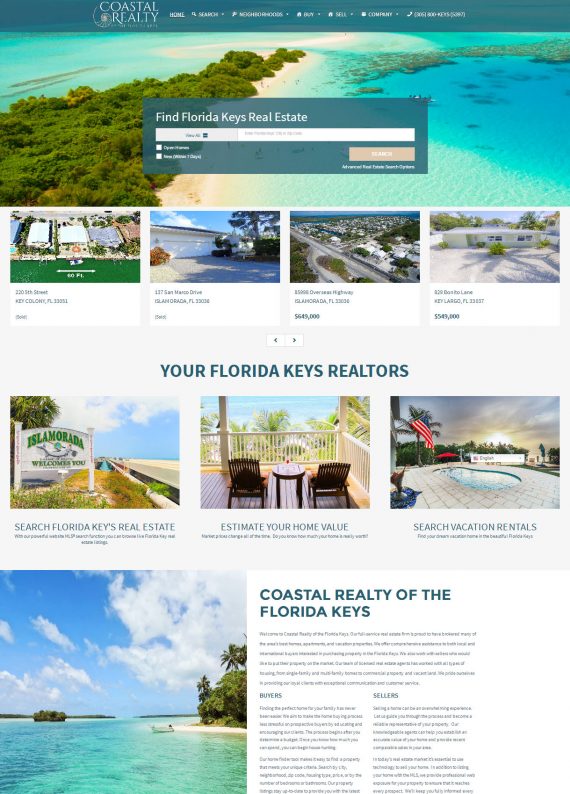At the top of the image, the text "Coastal Realty" sits against a stunning backdrop of crystal-clear blue water and sandy shores, encircled by a lush expanse of trees on a central island. Superimposed on this picturesque scene is the tagline "Fine Florida Keys Real Estate". Directly below, a series of home images are displayed: one features a substantial white garage, while another showcases a charming one-story home with a white roof and a palm tree in the foreground. In green text, it declares "Your Florida Keys Realtors", with an invitation to "Search Florida Keys Real Estate" positioned nearby. Adjacent to this section, an image captures two chairs on a balcony overlooking distant palm trees and serene waters. Beneath this, the text prompts "Estimate Your Home Value". To the right, an image highlights a swimming pool bordered by stone-paved surroundings and an American flag to the left, accompanied by the prompt "Search Vacation Rentals". Finally, the last box to the left revisits the stunning turquoise waters, sandy landscape, and trees, overlaid with the text "Coastal Realty of the Florida Keys". Below this, a main paragraph is followed by four smaller informational paragraphs, offering detailed insights.